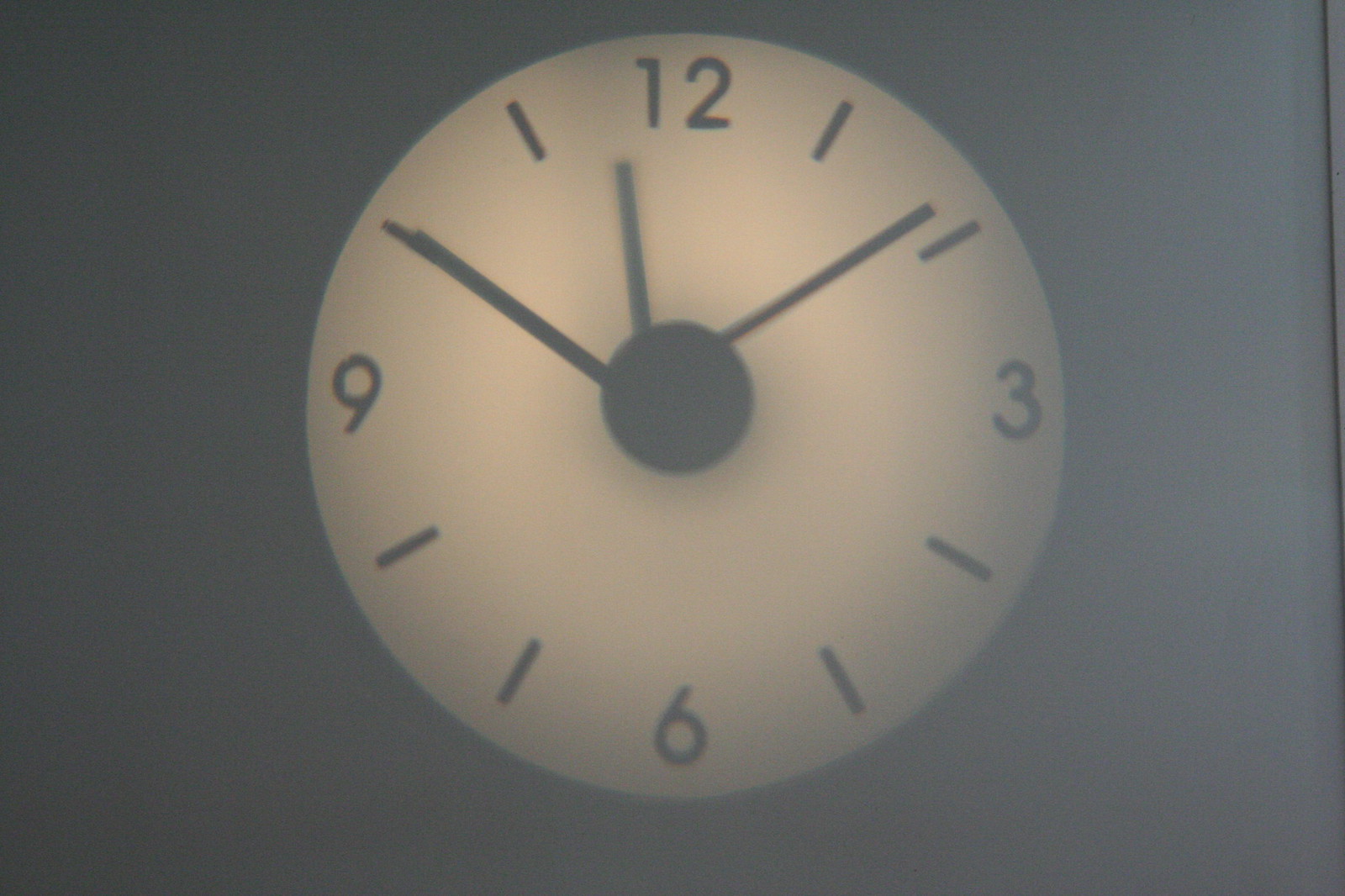This image depicts a clock with a somewhat surreal, almost video-game-like appearance. The clock face is white and features only the numbers 12, 3, 6, and 9, positioned at their respective intervals. The remaining hours are marked by simple tick marks. It has three black hands for hours, minutes, and seconds, all converging at a central black knob. The clock appears to display a time close to 10:10, with approximately 57 seconds. The photo itself is slightly blurred, making it difficult to determine the exact setting of the clock—whether it is mounted on a wall outside or inside a building. The backdrop of the image is black with a gray haze, adding to the mysterious and slightly indistinct quality of the scene. Additionally, the clock seems to be of an electric type that illuminates from the inside, despite the overall image appearing grayed out.